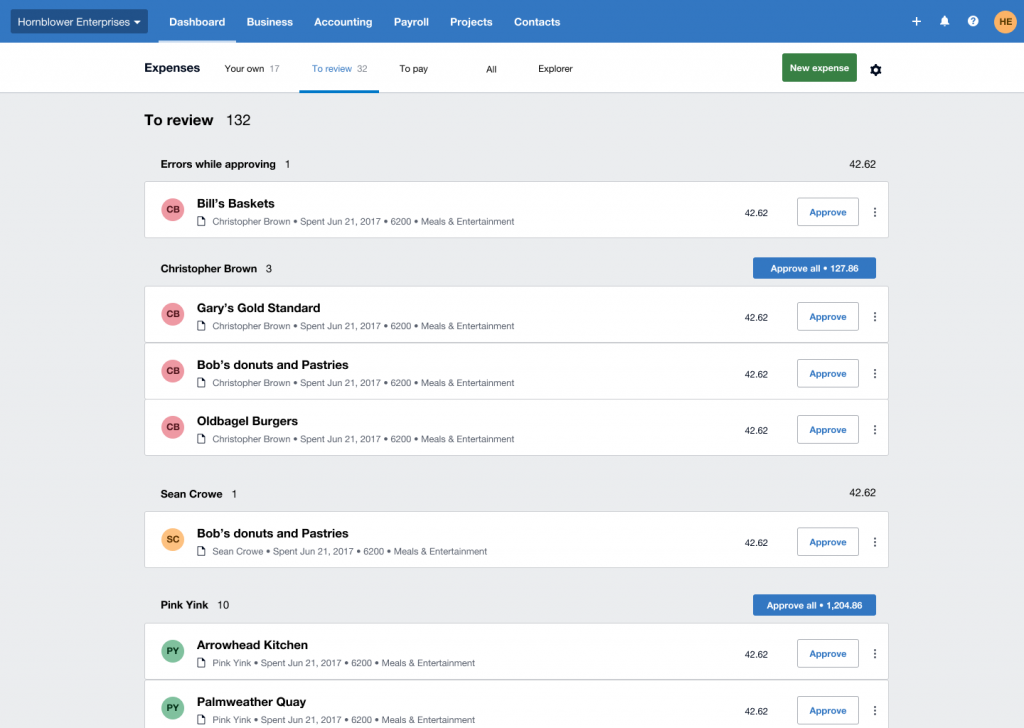The digital image appears to depict a user interface, likely from a business management software. This interface has a bright blue horizontal rectangular border at the top. Within a darker navy blue horizontal rectangle overlaid on the brighter blue border, there’s an indecipherable word followed by "Enterprises" in white font and a menu pull-down option. Adjacent to it, and continuing along the bright blue background, there are white font labels for various sections: Dashboard, Business, Accounting, Payroll, Projects, and Contacts. To the far right of this bar are several small icons.

Below this blue header, the main body on a white background prominently displays the word "Expenses" in bold black font. Adjacent to "Expenses" in regular black font is "your own" with the number 17. To the right, in blue font with a bold underline, "to review" is accompanied by the number 32. In black font again, subsequent labels read "to pay," "all," and "explore." On the right side, a green horizontal rectangle with white font states "new expense," with a settings icon next to it.

The rest of the page background transitions to an off-white or light gray color. At the top, in bold black font, it reads "to review" with the number 132. Below this is another bold black statement, "errors while approving," followed by the number 1. 

Continuing down, the page includes multiple horizontal sections with each entry containing a coral-colored circular icon bearing the initials "C-B" on the left side and a bold black font name next to it, such as "Bill's Baskets." Each entry appears to contain further unreadable text and numbers to the right. These sections are boxed with light gray outlines and feature a white rectangular area with the word "approve" in turquoise font. There is a light gray backgrounded section labeled "Christopher Brown" (corresponding to initials "C-B"), with a number 3 adjacent to it and a blue horizontal rectangular area that says "approve all" in white font.

Horizontal white rectangular sections follow, each starting with a coral circle containing "C-B." Names presented are "Gary’s Gold Standard," "Bob’s Donuts and Pastries," and "Old Bagel Burgers." Each has associated numbers like 42.62 and an "approve" box.

Further down, another section is highlighted with "Sean Crow" (bearing initials "S-C" in a yellow circle) and a gray area marked number 1. Entries for this section include "Bob’s Donuts and Pastries" and "Pink Yink," each with "approve" options. Finally, the bottom section includes "Arrowhead Kitchen" and "Palm Weather Quay" marked by a "P-Y" in a green circle.